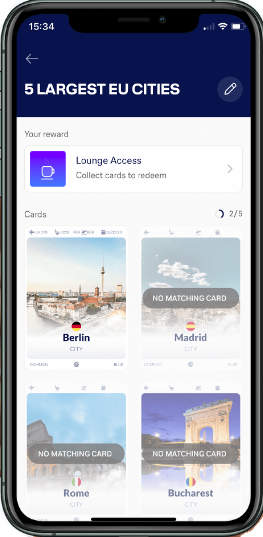In the image, a smartphone screen is displayed, showcasing a travel-themed app interface. At the top, a blue bar reads "Five Largest EU Cities," accompanied by back and edit buttons, the latter represented by a pencil icon. Below this header, the screen is divided into sections, each displaying one of four major European cities: Berlin, Madrid, Rome, and Bucharest.

Each city is represented by its name, national flag colors, and a corresponding image. Berlin is highlighted with the city's skyline and the Berlin flag symbol – a circle with black, red, and yellow bands. The Madrid section shows red and yellow colors and a grayed-out image labeled "No Matching Card." Similar labels appear on the sections for Rome (green, white, and red) and Bucharest. The Bucharest flag colors are indistinguishable due to image quality, appearing either green-yellow-red or blue-yellow-red.

At the center of the screen, a prominent "Your Reward" section details a prize of "Lounge Access," with instructions to "Collect Cards to Redeem." Further down, there is a card display section, where Berlin's card is fully visible, while the other cities show grayed-out cards with "No Matching Card" messages. On the side of the screen, a progress indicator reads "Two Out of Five," suggesting that two out of the five cards have been collected, although only four cities are currently displayed.